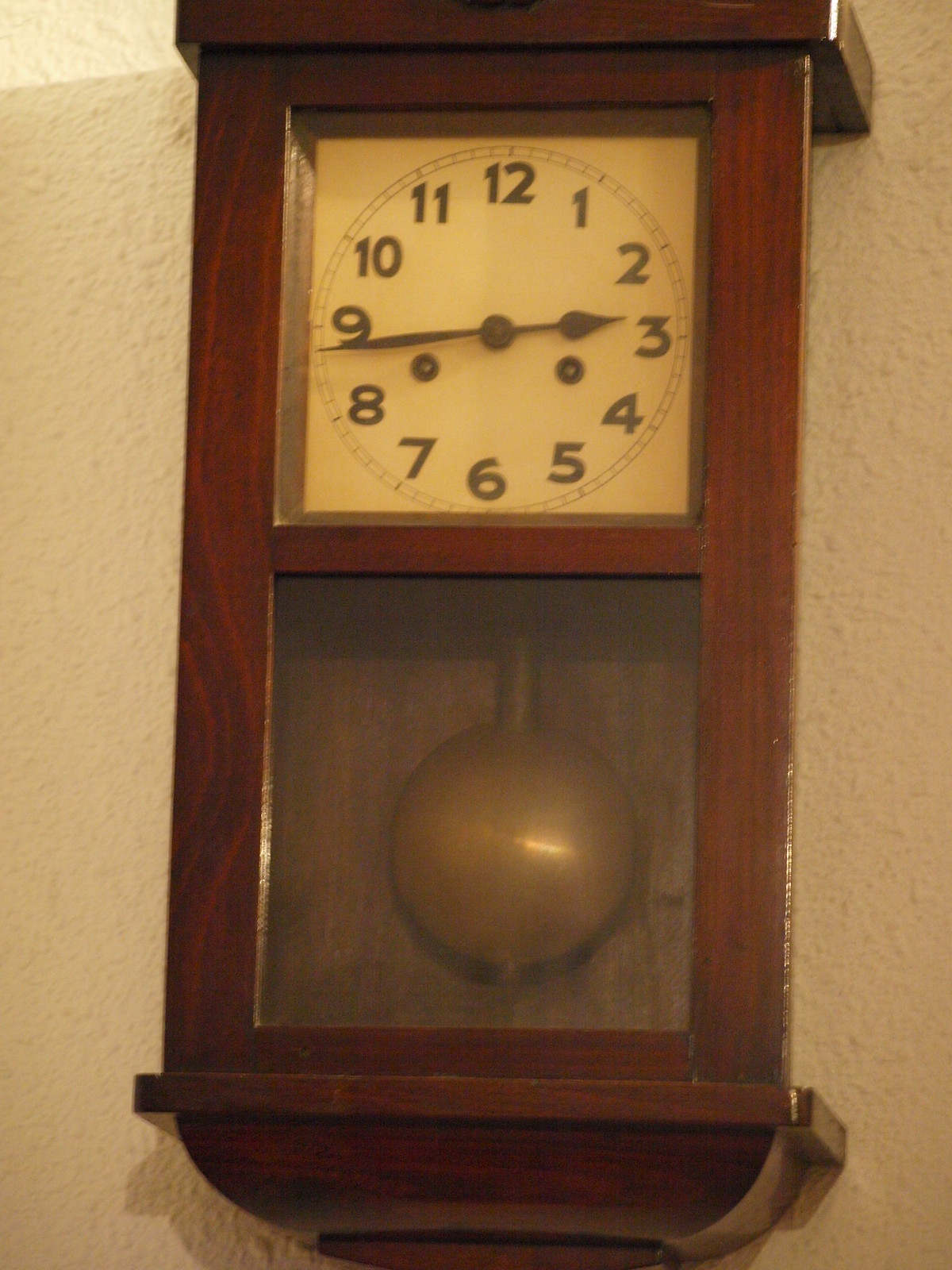The image depicts a wall clock mounted on an off-white, almost tan-colored wall that features a subtle, bumpy texture. The wall clock has a cherry wood exterior, characterized by a dark brown color with a hint of red. This clock has a traditional design and includes a pendulum, visible through a small glass window at the bottom, with the pendulum itself being golden-colored.

The clock face is square and has a yellow background, clearly showing the time as 2:44. The clock's hands are black and it has numerals from 1 to 12 in a clockwise arrangement, with small hash marks between each number to indicate individual minutes.